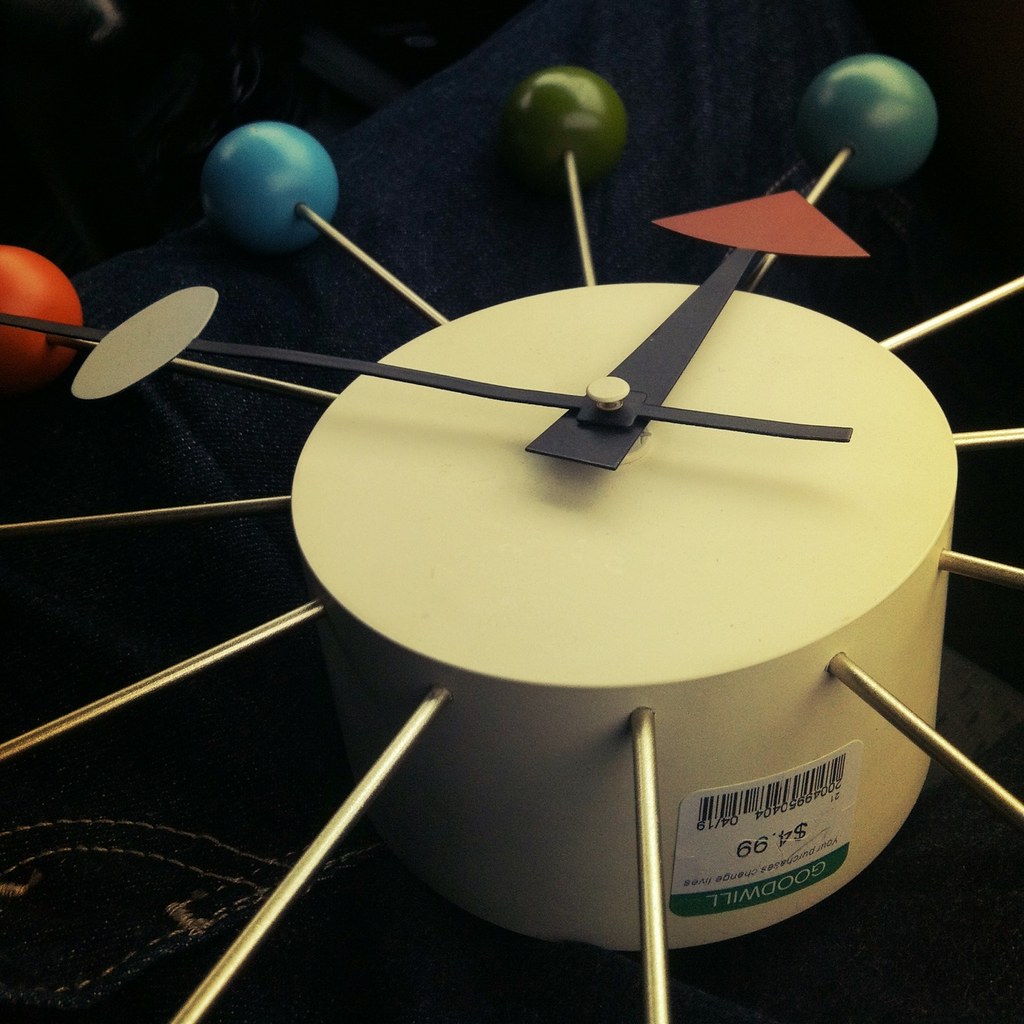This photograph features a highly unusual and artistic clock, viewed from an oblique angle, against an entirely black background. The clock itself has a vibrant yellow, somewhat cheeselike circular face, with prominent black minute and hour hands showing the time as quarter to twelve. The hour hand features a red diamond pointer, while the minute hand has a gold oval pointer. Radiating from the upper perimeter of the clock are bronze or golden metallic rods, each tipped with a distinctively colored ball. Visible in the image are a red ball, a blue ball, an army green ball, and a darker navy blue or green ball. Additional rods with balls extend out of the frame.

The clock is affixed with an upside-down label from Goodwill, marked $4.99 and featuring a barcode. It is placed on someone's lap, and the person is wearing blue pants. In the bottom left corner of the image, a metallic chain is partially visible. This clock merges functionality with a whimsical design, making it a striking timepiece.